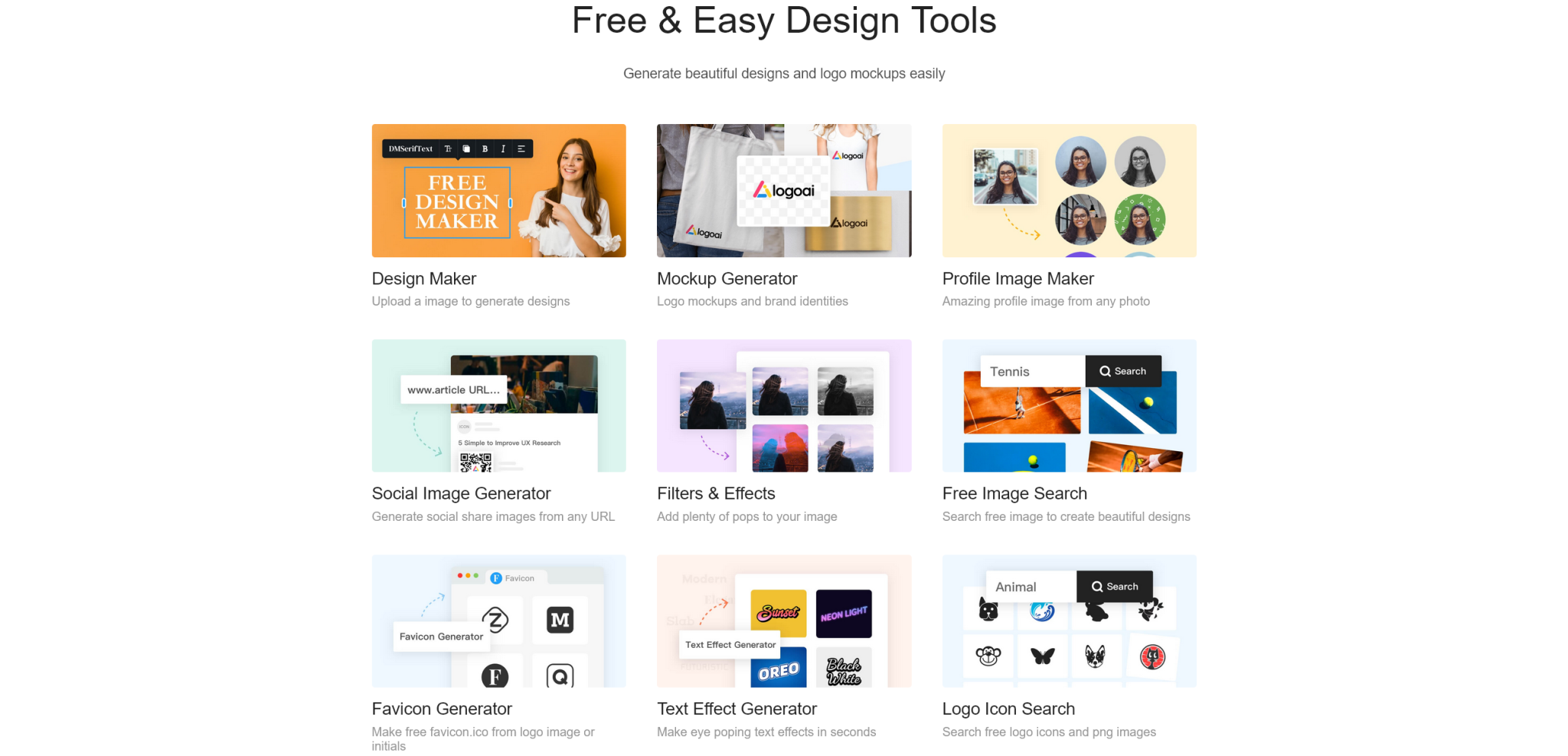Here’s a detailed and refined caption for the image:

---

The image showcases an advert for an online design platform. At the top, bold text reads "Free and Easy Design Tools," followed by a smaller subheading, "Generate beautiful designs and logo mock-ups easily." Beneath this, nine thumbnail images are displayed, each representing different features of the platform.

- The top-left thumbnail with an orange border features a woman in a white shirt pointing to her left at a blue box labeled "Free Design Maker." Above it, a black pop-up displays various design tools. Below, the text reads, "Design Maker: Upload an image to generate designs."
- Next to it, the thumbnail titled "Mock-up Generator" showcases a bag, a shirt, and a box, all printed with the logo "Logo AI."
- To the right, another thumbnail displays multiple images of the same woman, labeled "Profile Image Maker," with text below stating, "Amazing profile image from any photo."
- The second row starts with the "Social Image Generator" thumbnail.
- Followed by "Filter and Effects," showcasing the platform’s filtering options.
- And then "Free Image Search," indicating a search feature for images.
- In the third row, the leftmost thumbnail is titled "Favicon Generator."
- Next to it is the "Text Effect Generator."
- The final thumbnail to the right is "Logo Icon Search."

Each thumbnail is designed to highlight the platform’s diverse and user-friendly design tools, making it easy for users to create stunning visual content effortlessly.